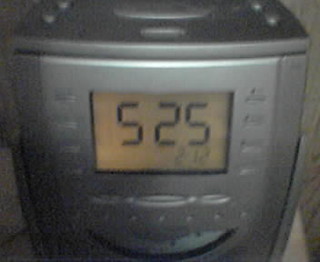This photograph showcases a somewhat blurry yet intriguing image of a vintage CD player. The device, likely from an earlier era of digital music, features a compact design with a clearly visible digital screen displaying the numbers "525." Just below this, towards the bottom right corner of the screen, the numbers "212" are faintly discernible. The CD player is equipped with multiple buttons, arranged thoughtfully to aid user operation. Dominating the top of the device, a prominent central button likely serves to eject the CD tray, indicative of its key functional role. Flanking this central button, two smaller buttons are situated symmetrically, possibly used for play, pause, or track navigation. The aged charm of the CD player is palpable, evoking a sense of nostalgia for the early days of digital music.